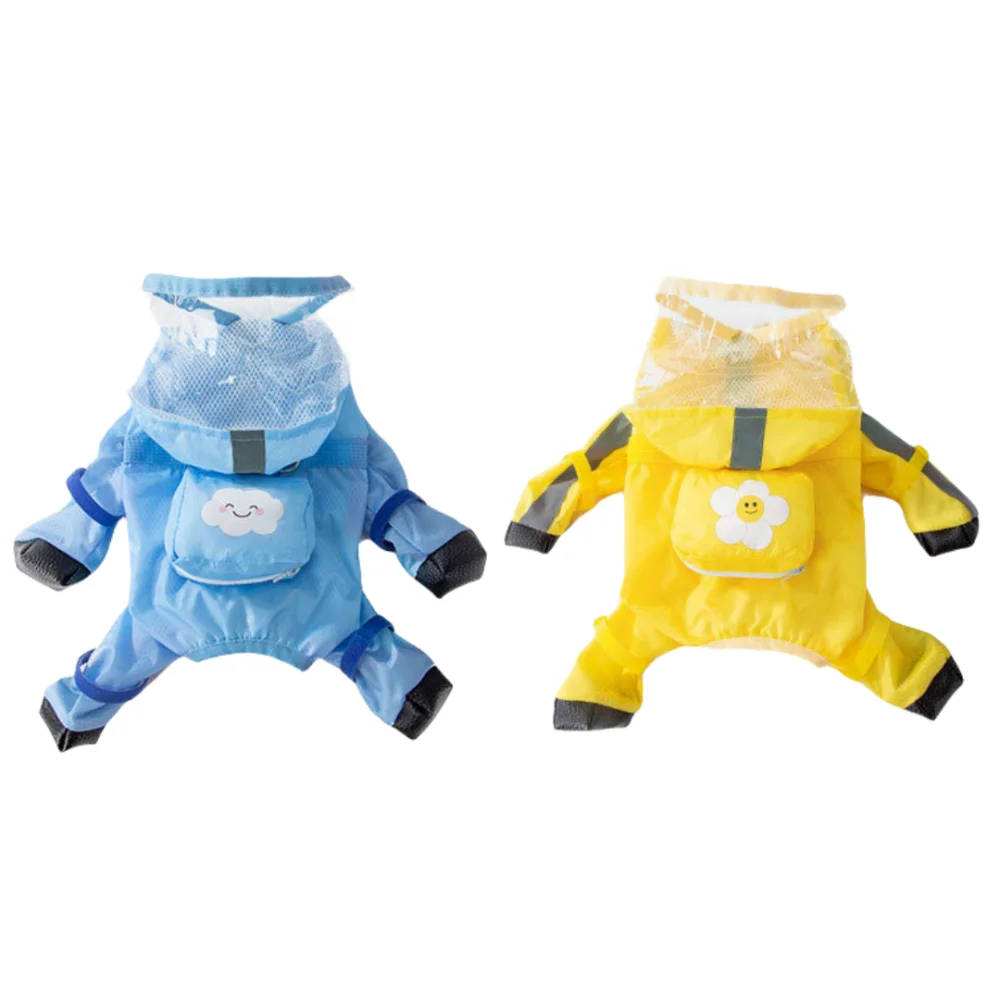In this image, we see two infant outfits designed to resemble miniature hazmat or beekeeper suits, likely for babies aged three to six months. The outfit on the left is predominantly light blue with dark blue trimmings, while the one on the right is mainly yellow with black trimmings and a dark stripe. Both suits feature mesh-netted headpieces, which resemble hoods folded back, adding to their hazmat or beekeeper-like appearance. Each suit has a distinctive patch on the chest area: the blue suit has a white, smiling cloud with closed eyes and red cheeks, and the yellow suit has a white daisy with a smiling face in its yellow center. The suits also have black tips on the edges of the sleeves and legs, contributing to their detailed, thematic design.